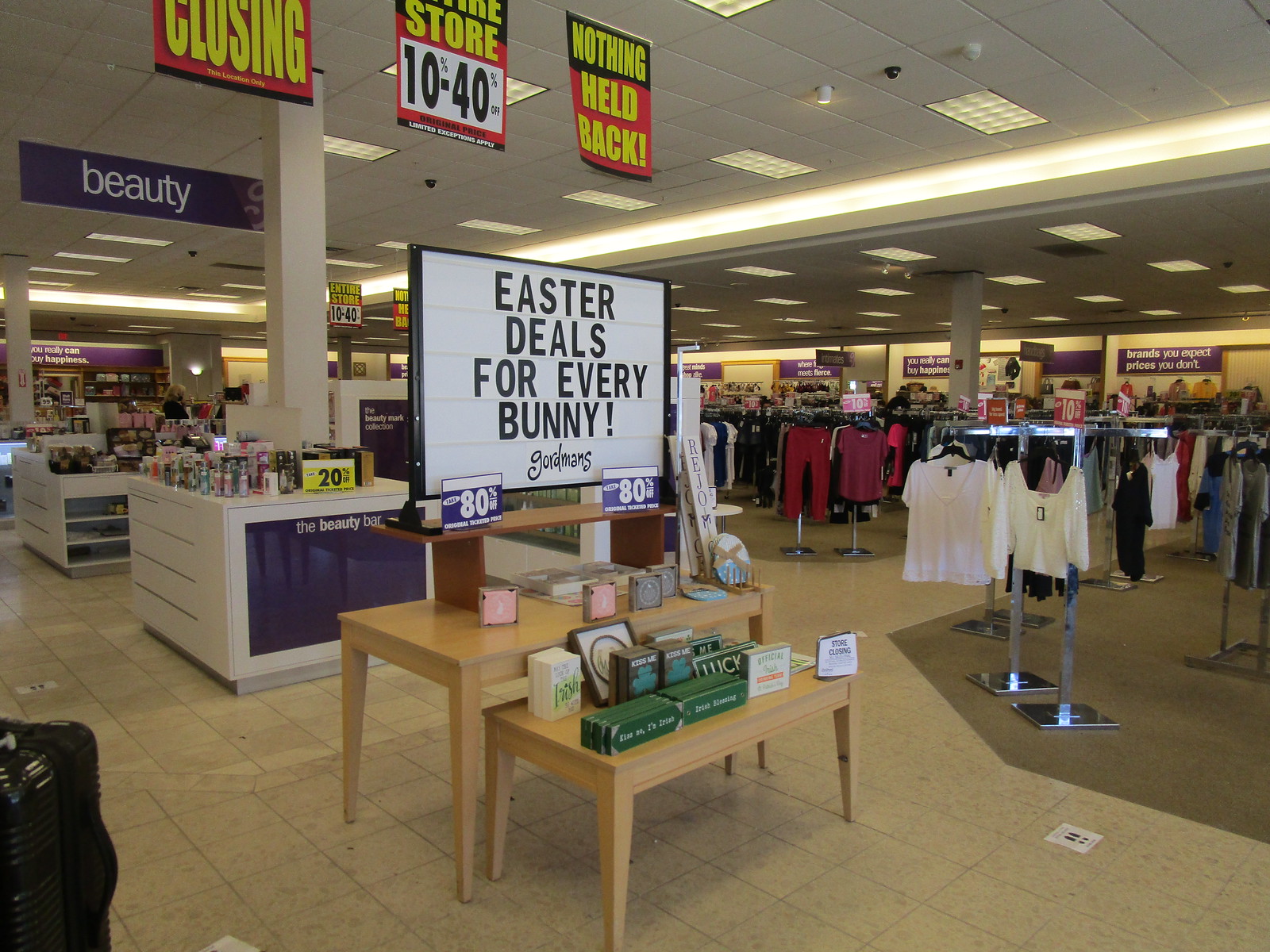This detailed photograph captures the interior of a Gordman's clothing store. Prominently featured in the center is a large white sign with black letters that declares "Easter Deals for Every Bunny," followed by "Gordman's" beneath it, flanked by a smaller 80% off notice in white font on a purple background. Below the sign are two light wood-colored tables, one slightly taller than the other, adorned with St. Patrick's Day decorations in various shades of green. Surrounding these tables is a variety of women's apparel in colors such as white, burgundy, red, blue, gray, and pink, displayed on racks. The image is taken from the edge of an aisle, which branches off to the right, revealing a mix of flooring: tile on the left and carpet on the right. The store is lit by overhead fluorescent lights and features encased lighting on the ceiling. In the background, signs hint at the store’s closing, with messages such as "Nothing Held Back" and "Closing," partially visible above an area identified as the register and counter, adorned with an additional sign reading "Beauty." The store layout and fixtures, including the glimpse of a black shopping cart's edge in the left-hand corner, add to the vivid depiction of the setting.